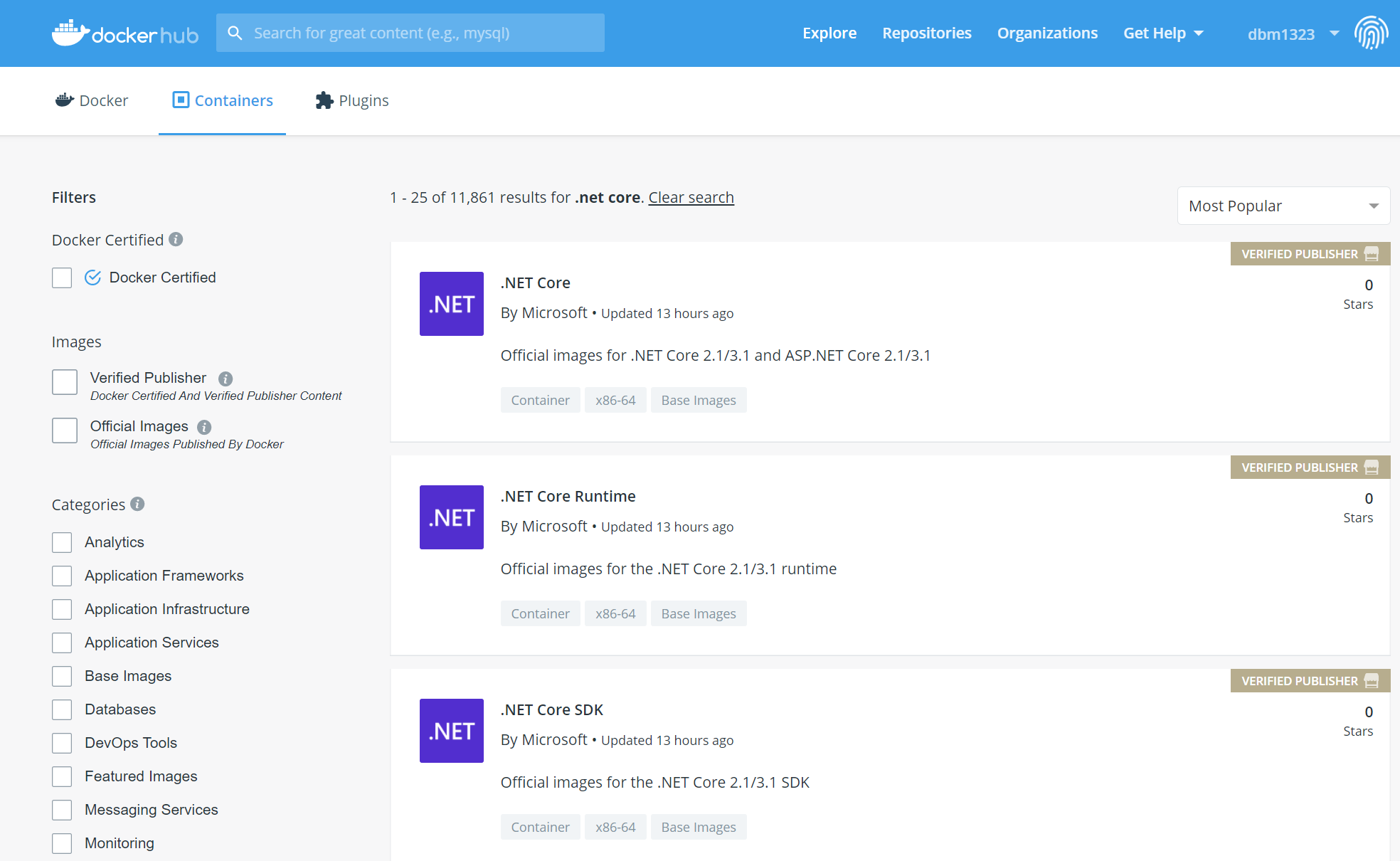This image is a detailed screenshot of Docker Hub's user interface. At the top, the Docker Hub logo is prominently displayed, featuring a stylized whale with shipping containers on its back, symbolizing containerized applications. Below the logo, the main navigation bar includes options such as "Search for great content," "Explore," "Repositories," "Organizations," and "Get Help."

To the left of the interface, there is a sidebar with various filter options, including categories such as "Docker-Certified Images," "Verified Publisher," and "Official Images." The Categories section is extensive, listing options such as "Analytics," "Application Frameworks," "Application Infrastructure," "Application Services," "Base Images," "Databases," "Development Operation Tools," "Featured Images," "Messaging Services," and "Monitoring."

Three specific items are highlighted within the search results: 

1. **.NET Core**: 
   - Listed as "Official Images for .NET Core 2.1 and 3.1, and ASP.NET Core 2.1/3.1." 
   - It has no user reviews or stars.

2. **.NET Core Runtime**: 
   - Described as "Official Images for the .NET Core 2.1/3.1 Runtime."
   - This category also has no user reviews or stars.

3. **.NET Core SDK**: 
   - Marked as "Official Images for the .NET Core 2.1/3.1 SDK."
   - Similarly, this category appears with zero reviews or stars.

The screenshot provides a comprehensive view of Docker Hub's robust functionality and extensive categorization, though the specific search results for .NET Core tools have not yet been reviewed or rated by users.